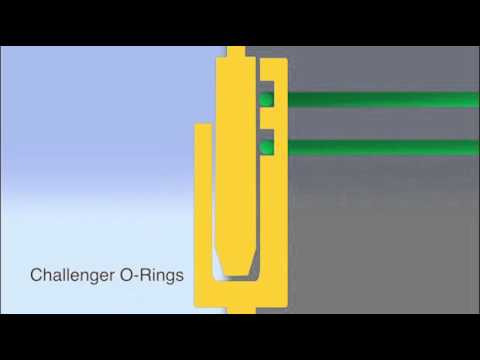This is a detailed illustration featuring the Challenger O-Rings. The image is letterboxed with black bars on the top and bottom, suggesting it might be a slide or a screenshot. On the left side, there is a light bluish to magenta rectangle that reads "Challenger O-Rings" in black font. The center of the image is dominated by a yellow device or connection unit with two parts: a yellow rectangle and a U-shaped yellow clamp. The right side has a dark gray background with two horizontal green rods that appear to lock into the yellow connection unit. The overall composition is structured to highlight the interplay between the parts and their respective colors for clear visual distinction.